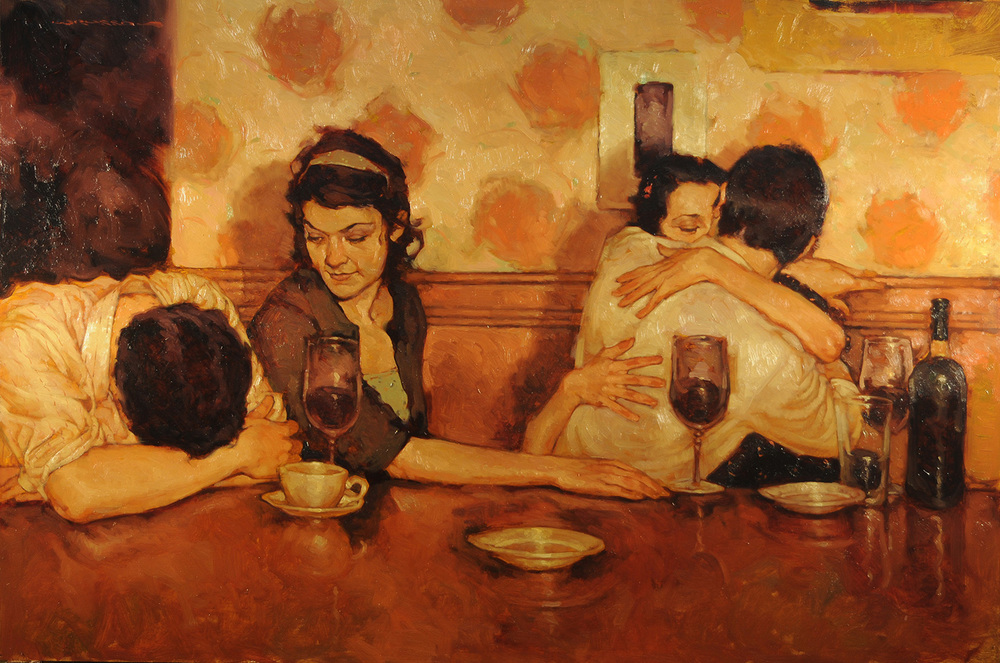This oil painting, reminiscent of a 1950s style, portrays an intimate scene at a restaurant table featuring two couples. The table, a warm orangish-brown wood, is set in a cozy booth with a retro wallpaper backdrop adorned with light yellow and orange circular flowers. The right side of the painting captures a romantic moment where a man with dark brown hair in a white shirt passionately kisses a woman with brown hair, whose right eye and upper face are visible with eyes seemingly closed. Her arms are wrapped around him, adding to the tender embrace.

In striking contrast, the left side depicts a more somber scene. A man, also with brown hair and wearing a white shirt rolled up to his elbows, has his head down on the table, appearing tired or despondent. Beside him, a woman with short brown hair and a gray headband looks down at him with a gentle smile, her right forearm resting on the table. Both couples have scattered tableware in front of them: wine glasses with remnants of purple wine, a green wine bottle, a coffee cup with a saucer, and possibly a water glass.

Above the embracing couple, a small painting hangs on the wall, adding to the nostalgic ambiance. The entire scene, bathed in hues of yellow, orange, and hints of gray, evokes a feeling of a late-night gathering where emotions, both joyous and melancholic, are shared.